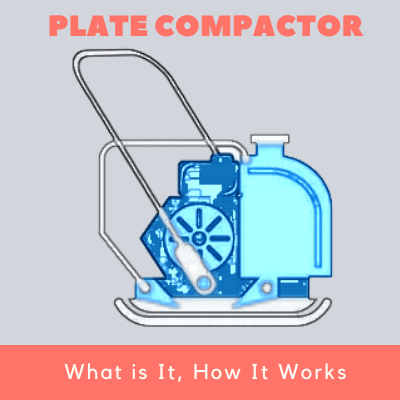The image is an informational graphic showing a detailed line drawing of a plate compactor, a machine used for compacting surfaces. The background is gray, with the title "PLATE COMPACTOR" prominently displayed at the top in capitalized red letters. The drawing features a light blue plate compactor with a distinctive flat, sled-like metal base that curves at both the front and back. Attached to the base is a large handle resembling that of a lawnmower, designed for manual operation. Central to the device is a light blue component resembling a large gas tank with a white cap, suggesting engine-powered functionality. To the left of the gas tank, there is a darker section that possibly represents a motor or gear mechanism. At the bottom of the image, against a red rectangular background, white text poses the questions "What is it?" and "How it works?" although no further explanatory information is provided within the graphic itself.